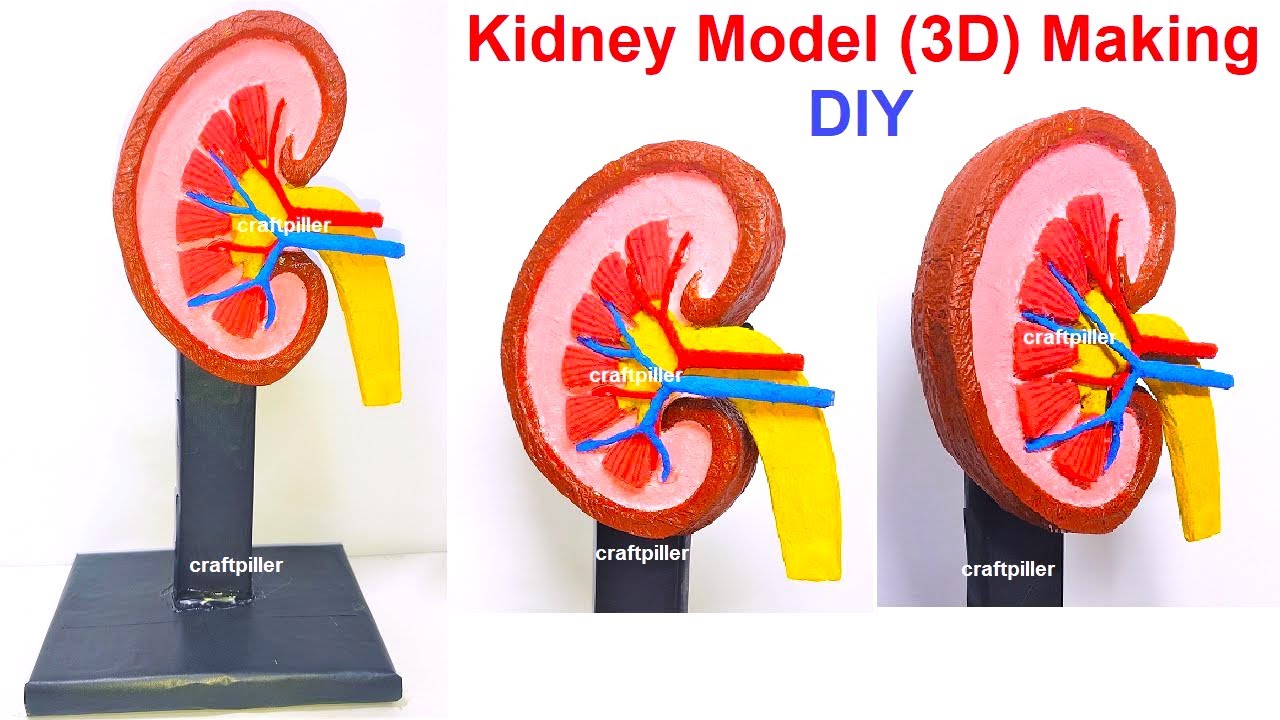The image showcases a plastic 3D model of a kidney displayed in three separate panels, each offering a different angle of the same model. The text at the top of the image reads "Kidney Model 3D Making" in red, followed by "DIY" in blue. This cross-sectional kidney model is mounted on a green or gray stand with a supporting gray piece to elevate it. The kidney itself is pink at the center with a red border and features five thick red splotches positioned in a crescent formation. Interspersed between the splotches are red and blue lines representing veins and arteries, and a thicker yellow pipe-like structure extends downward, likely depicting the ureter. The brand name "Craft Pillar" is prominently displayed in white text on both the kidney and at the bottom of the panels. Each panel provides a slightly different perspective, showing the intricate details and coloring of the model from various angles.